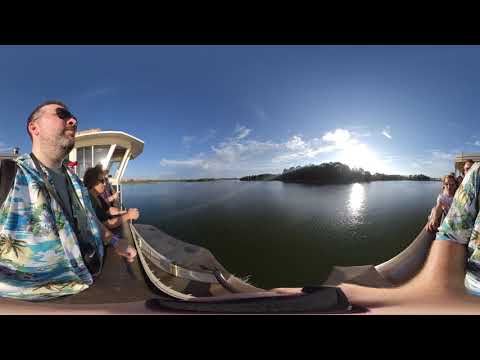This detailed photograph, captured with a fisheye lens providing a 360-degree panoramic view, depicts a serene scene at the edge of a lake or river. The water is calm, displaying muted shades of green and blue, and is surrounded by a shoreline lush with trees. Overhead, the sky is a bright blue adorned with a few wispy white clouds through which the sun occasionally peeks, casting a bright, natural light on the scene.

In the foreground, several people are standing on the edge of a dock, leaning on the balcony railing and admiring the tranquil water. Prominent among them is a tall Caucasian man, closest to the camera, wearing black sunglasses and a Hawaiian shirt featuring a white background with beach scenes, including palm trees, sand, and water. His shirt, partially unbuttoned over a gray t-shirt, includes a mix of blue and yellow colors. He has a very serious expression as he gazes out over the water. Beside him stands a woman also donning sunglasses; her arms rest casually on the railing as she takes in the view, and she is dressed in a dark-colored shirt.

On the left side of the dock, there is a glass structure with white trims that appears to be some kind of lookout. The overall environment suggests a leisurely moment shared by people appreciating the natural beauty around them, with the bright, inviting atmosphere complemented by the vibrant attire of the observers.